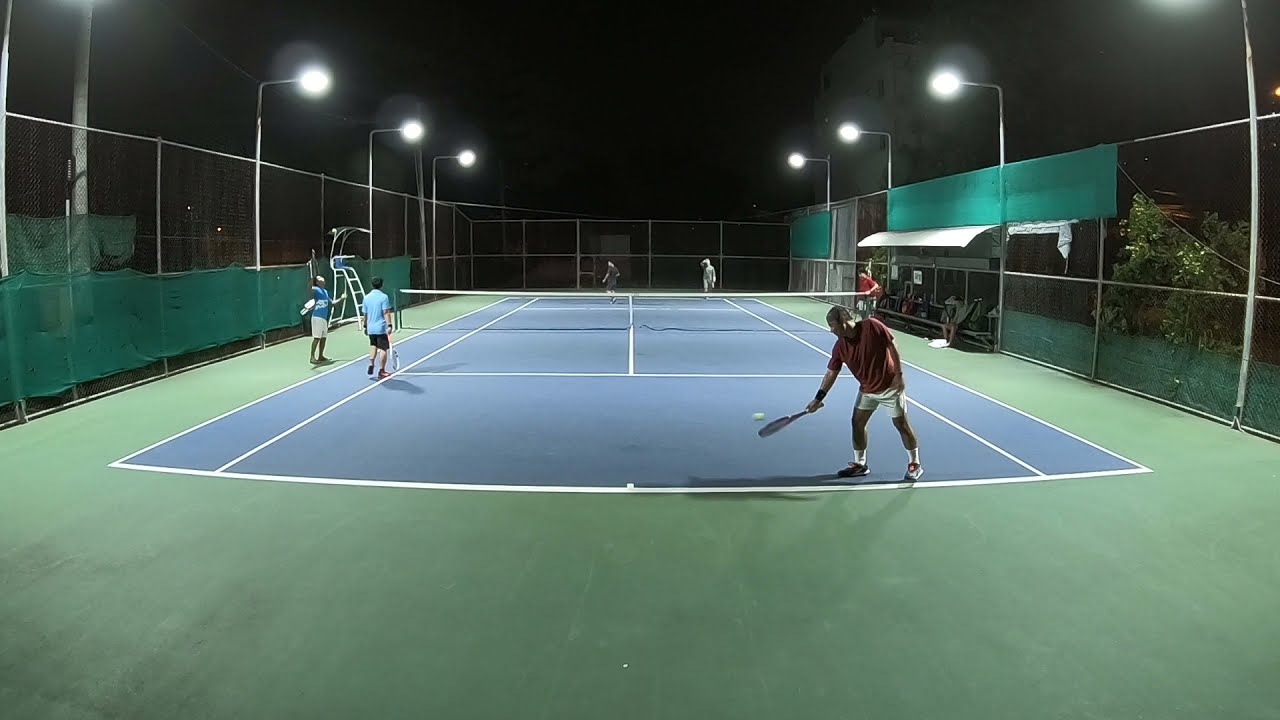The image depicts an outdoor tennis court illuminated by multiple circular lights against a black, nighttime sky. The central playing area of the court is blue with white boundary lines, while the surrounding edges are green. The court is encased by a chain link fence adorned with green see-through panels. On the court, six people are engaged in a match. Positioned on the right is a player in a tan shirt, white shorts, and black-and-white shoes, seemingly about to serve. To the left of the court, two players stand, one donning a light blue shirt with black shorts and the other in a dark blue shirt with white shorts. In the background, a man dressed in a black shirt and black shorts is visible. Additionally, there is a red-shirted participant on the right near a bench and a canopy, suggesting an area where players have placed their belongings. The court is well-lit with a series of lights, ensuring clear visibility for the nighttime game.